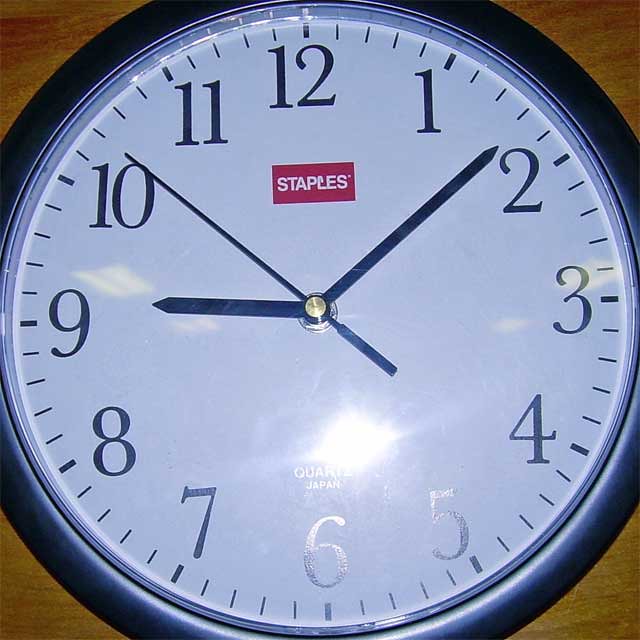This image prominently features a clock that occupies the central area, while the corners reveal glimpses of a brown table. The clock's outer rim is a light blue hue, contrasting with its white face. Black numerals mark the hours, accompanied by small black lines denoting the minutes between them. The clock's hands, also black, are positioned to indicate the time as 9:08. Notably, beneath the number 12, there's a red rectangle emblazoned with the word "Staples." Above the number 6, the words "Quartz" and "Japan" are inscribed. Additionally, there's a visible reflection of the camera's flash located near the 6.